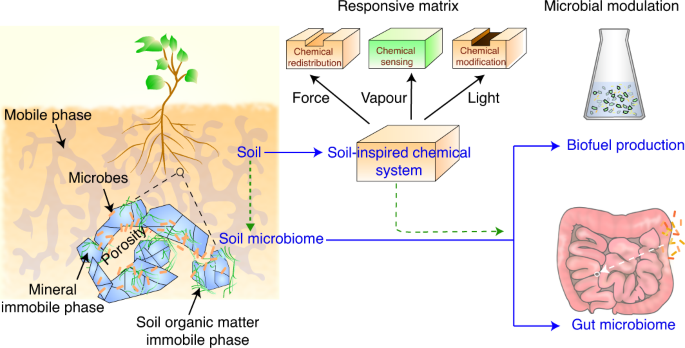The diagram intricately illustrates the interaction between plants, soil, and chemical processes within a soil-inspired chemical system. On the left-hand side, a detailed sketch of a plant reveals its roots embedded in soil, encapsulating the "mobile phase" with downward arrows pointing to "microbes," "porosity," and "soil organic matter immobile phase" beneath the earth. The "mineral immobile phase" is also marked within this underground section. Centrally, the diagram highlights a "responsive matrix" heading above three interconnected boxes labeled "chemical redistribution," "chemical sensing," and "chemical modification." These processes are influenced by "force," "vapor," and "light," depicted with respective arrows. A pivotal "soil-inspired chemical system" box anchors the central schema. On the right-hand side, a beaker labeled "microbial modulation" sits atop, with arrows leading downwards to "biofuel production" and further to an image of intestines, denoting the "gut microbiome." This right-hand sequence underscores the transformation from soil components to energy solutions and biological systems within the gut.